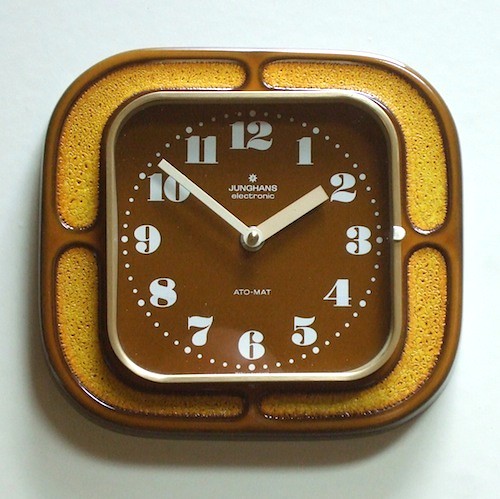This color image showcases a distinctly 1970s-style wall clock mounted on a plain gray background. The clock features a unique design with a central circular face encased in a brass square, which is itself contained within a larger brown square adorned with four boomerang-shaped yellow sections that give a sponge candy or melba toast-like appearance. The clock face is brown, displaying gray numbers from 1 to 12, with corresponding gray minute dots encircling it, and is marked with a gray minute hand and hour hand. The brand name "Jung Hand Electronic" is inscribed below the "12," and below the clock hands, it reads "ATO-MAT." The overall aesthetic, with its gold, brown, and brass components, evokes a vintage 1970s charm.